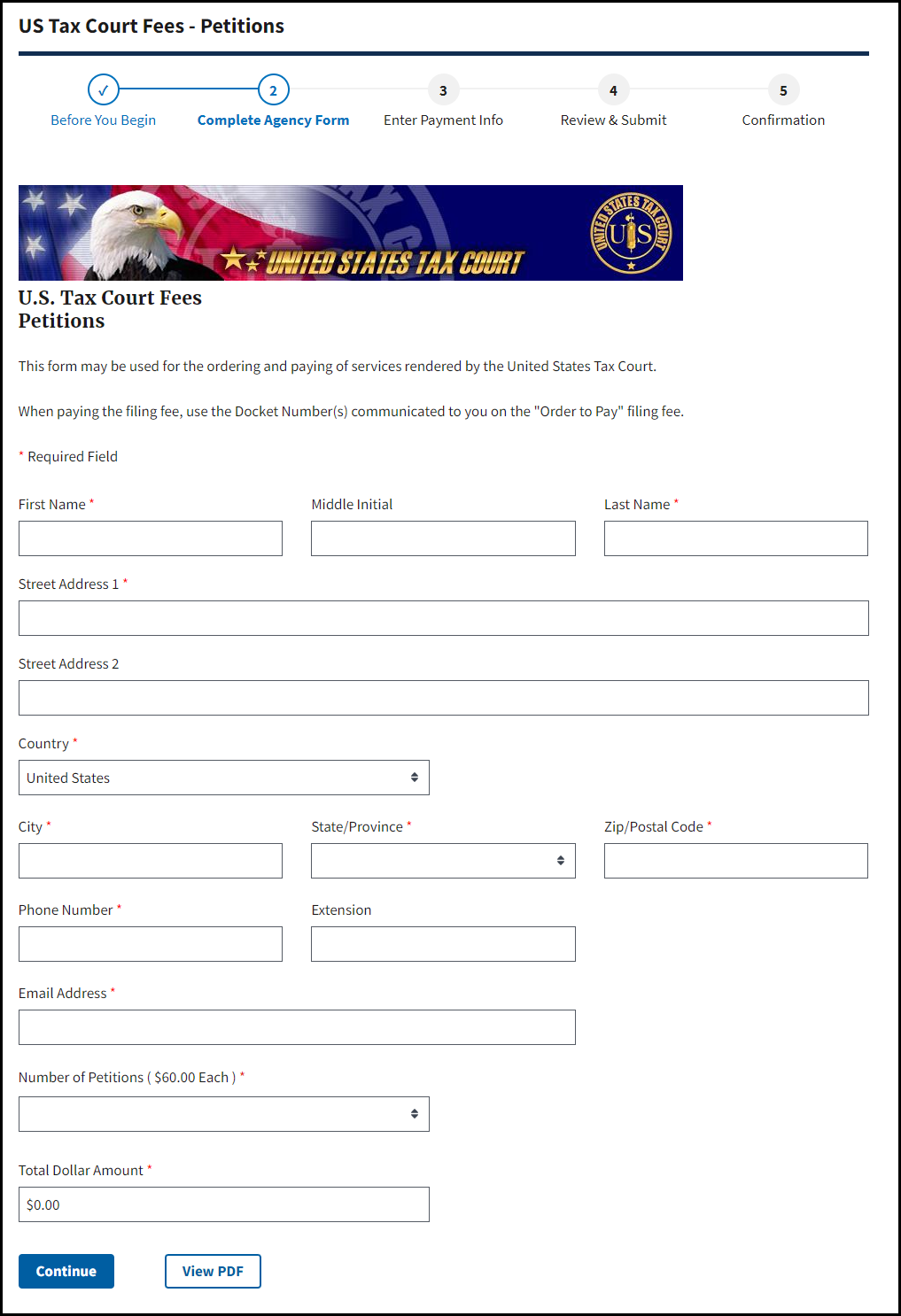This image is a detailed screenshot of a U.S. Tax Court Fees Petitions website form. At the top, a structured progress bar guides users through five steps: "Before You Begin" with a check mark, "Complete Agency Form" highlighted in a blue circle with the number 2, followed by grayed-out steps "Enter Payment Info," "Review and Submit," and "Confirmation." Below the progress bar, a prominent header features an eagle in front of an American flag, flanked by gold stars. The text "United States Tax Court" is displayed in gold in the center, with a circular U.S. Tax Court logo to the right.

The form itself is designed to facilitate the ordering and payment of services rendered by the United States Tax Court. Specific instructions indicate that when paying the filing fee, users should utilize the docket numbers provided in the order to ensure accurate processing. Various fields on the form are marked as required, such as first name, last name, street address 1, country (prefilled to the United States), city, state/province, zip/postal code, phone number, email address, number of petitions ($60 each), and the total dollar amount. There is also an optional field for street address 2 and an extension field for phone numbers. At the bottom of the form, two buttons are presented: a blue "Continue" button and a white "View PDF" button.